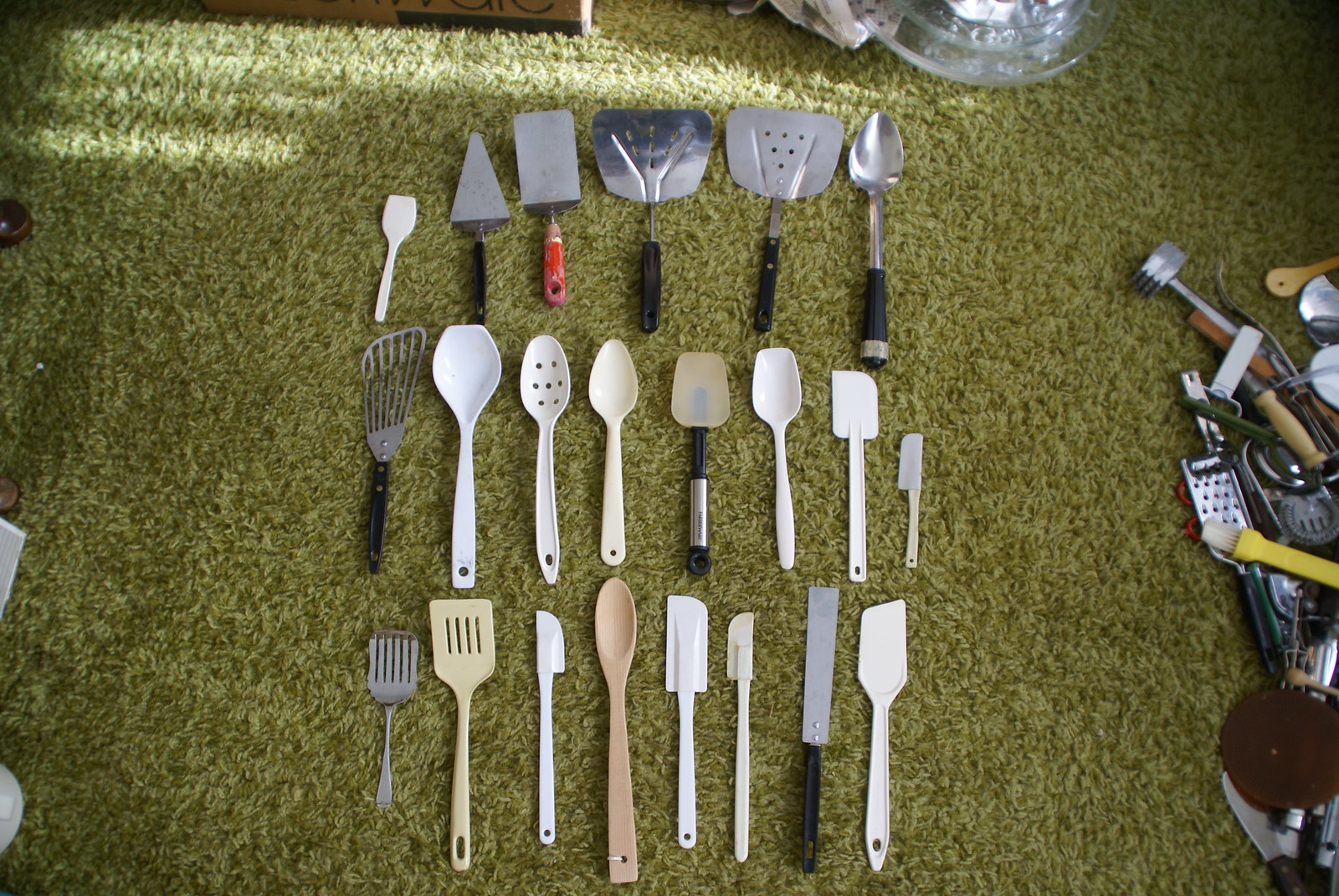In this vibrant interior photograph taken from above, the viewer's eye is drawn to a green shag carpet floor bathed in sunlight streaming into the room. Neatly arranged on the green carpet are three horizontal rows of various kitchen utensils, predominantly spatulas and spoons, but also including forks, strainers, and graters. The top row features six utensils, including a mix of white and black spatulas, a red-handled metal spatula, and a black-handled metal spoon. The second row displays eight utensils, showcasing diverse designs such as a black-handled metal spatula with perforations, a white spoon with seven holes, and multiple white spatulas. The bottom row also consists of eight utensils, ranging from a line-holed metal spatula to a tan plastic spatula and a wooden spoon. Off to the side, a clutter of additional kitchen equipment, including more spatulas and a grater, is visible, adding to the detailed array of culinary tools.